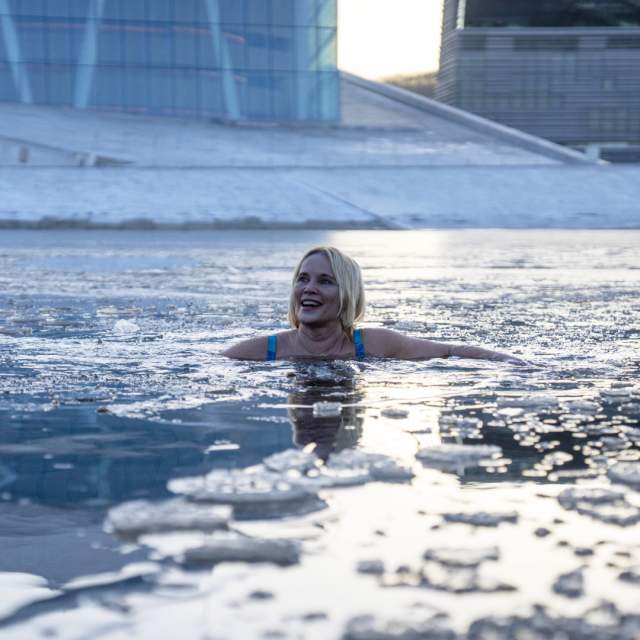The colour photograph captures a blonde-haired woman bathing in an icy body of water, her head and shoulders visible above the surface, which is filled with floating chunks of white ice. The pale-skinned woman, wearing a blue bathing suit with visible straps on her shoulders, has relatively short, chin-length hair with dark roots and is laughing while looking up to her left. The scene has a cold colour palette dominated by blues, whites, and blacks. Surrounding her are blurry but distinguishable large buildings, with a sloped, snow-covered area leading down to the icy water. Sunlight filters through the background, adding a bright contrast to the otherwise cool tones. The woman is centrally positioned in the image, which has no other people or objects in view, highlighting her solitary plunge into the frigid water.